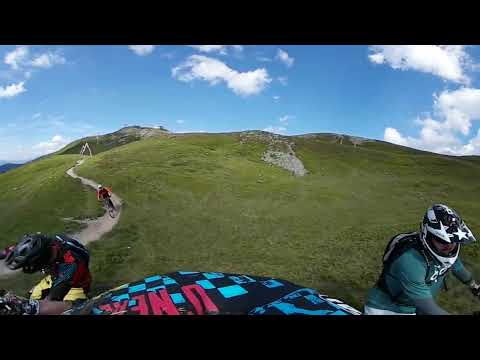The image appears to be captured from a GoPro camera mounted on a helmet, providing a first-person perspective from a bicycle or off-road motorcycle. Below the camera’s vantage point, a rounded rim with a black and teal checkered pattern and red lettering indicates the presence of the helmet. The scenery features a low-lying, grassy mountain with a distinctly hilly terrain. A winding dirt path is visible on the left side of the image, where a person in a red shirt is biking downhill toward the camera. In the near foreground, two other cyclists are present: one on the left wearing a black helmet, possibly riding a yellow bike or wearing yellow trousers, and one on the right sporting a black and white helmet adorned with a white star, dressed in a green shirt and protective gear. The sky is bright blue with a few puffy clouds scattered, adding a slight contrast. Notably, the image is bordered by black at the top and bottom, and the fisheye effect of the lens slightly warps the overall view, emphasizing the dynamic and adventurous off-road activity captured on the grassy hillside.